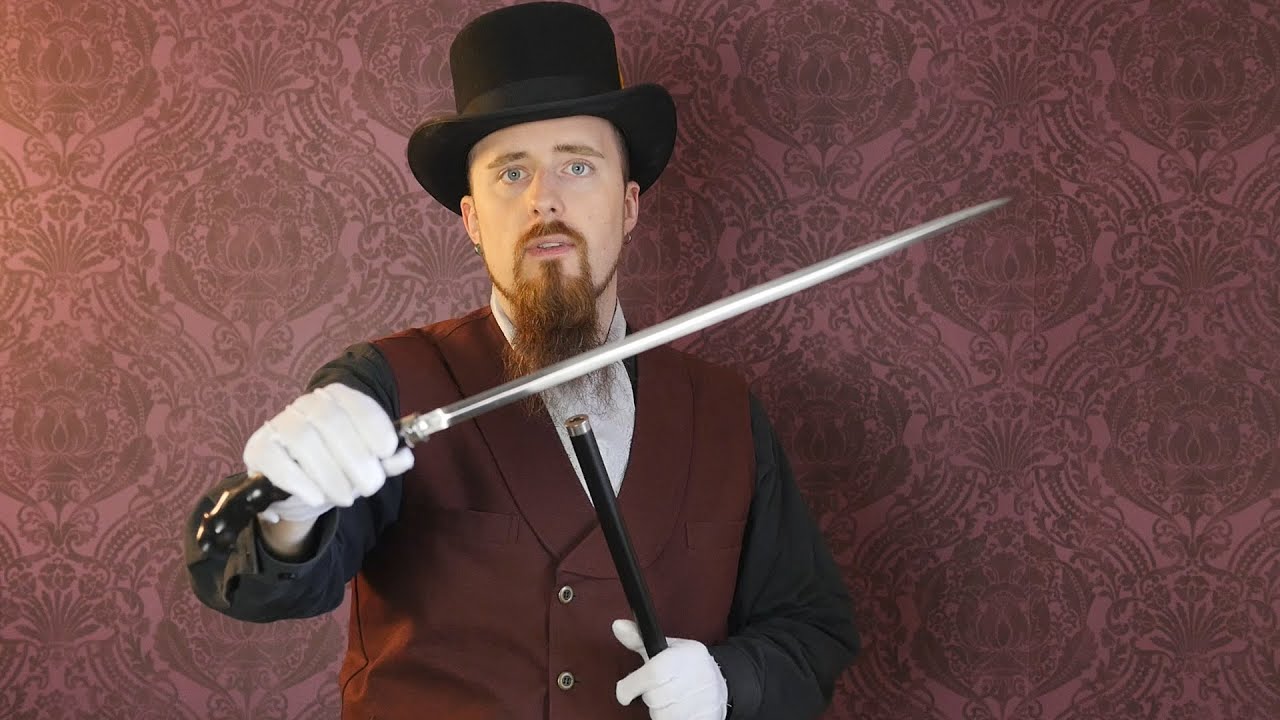The image depicts a gentleman who resembles a stage magician or a role player posing in front of an ornate, maroon velvet-patterned wall. He is a white man with a neatly kept, long reddish-brown goatee and mustache, and piercing blue eyes. On his head, he wears a black top hat. His attire includes a unique shirt that has a white collar and chest portion, black sleeves, and an overlay of a dark, reddish-brown vest with buttons. Around his neck, he sports a cravat or neckerchief, adding a touch of old-world charm. He is also adorned with white gloves, maintaining an elegant appearance. In one hand, he holds a saber, its blade glinting as it's unsheathed, while the other hand grips the sheath. The overall scene suggests a theatrical or magical setting, with the gentleman presenting the saber, possibly as part of a performance or trick.